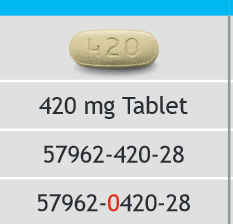The image features a simple but detailed layout. At the very top of the image, there's a thin blue line running horizontally. Directly beneath this blue line, there is a clear image of a small, white, oval-shaped tablet. This tablet prominently displays the inscription "L20" in black lettering at its center.

Below the image of the tablet, the text "420 MG tablet" is written in black and is separated from additional information by fine white lines. The subsequent section contains the string “57962-420-28” in black letters and numbers.

Following another white line, there is a final string “57962-0420-28,” where most of the characters are black except for a red zero. Thus, the sequence reads: “57962- red zero -420-28.” 

Additionally, there appears to be a vertical grayish line running down the side of the image, indicating an area to scroll through the image content.